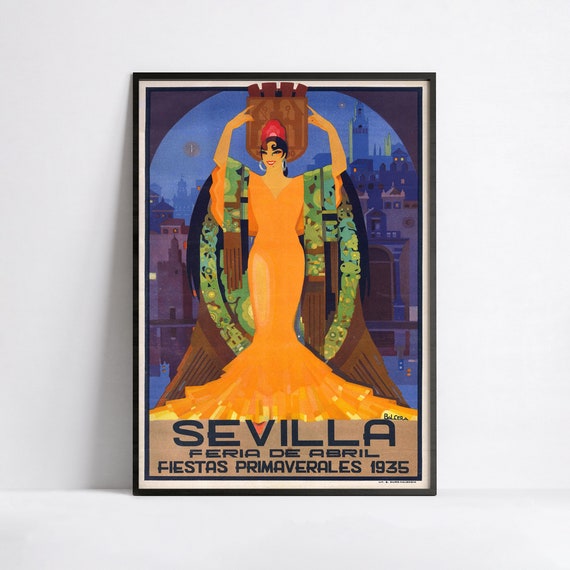This image depicts a vintage Art Deco-style poster from 1935 entitled "Sevilla Feria de Abril Fiestas Primaverales." The vibrant poster, set against a white wall and framed in black, features a striking woman as its central figure. She is adorned in a floor-length orange dress with a shawl of green and blue hues draped over her arms. Her arms are elegantly raised above her head with her index fingers pointing upwards towards a red headdress. She completes her look with large hoop earrings and a radiant smile. The backdrop reveals a dimly lit twilight cityscape of Seville, with its characteristic buildings and high-rises presented in shadowy blue and purple tones, enhancing the poster's old-world charm.